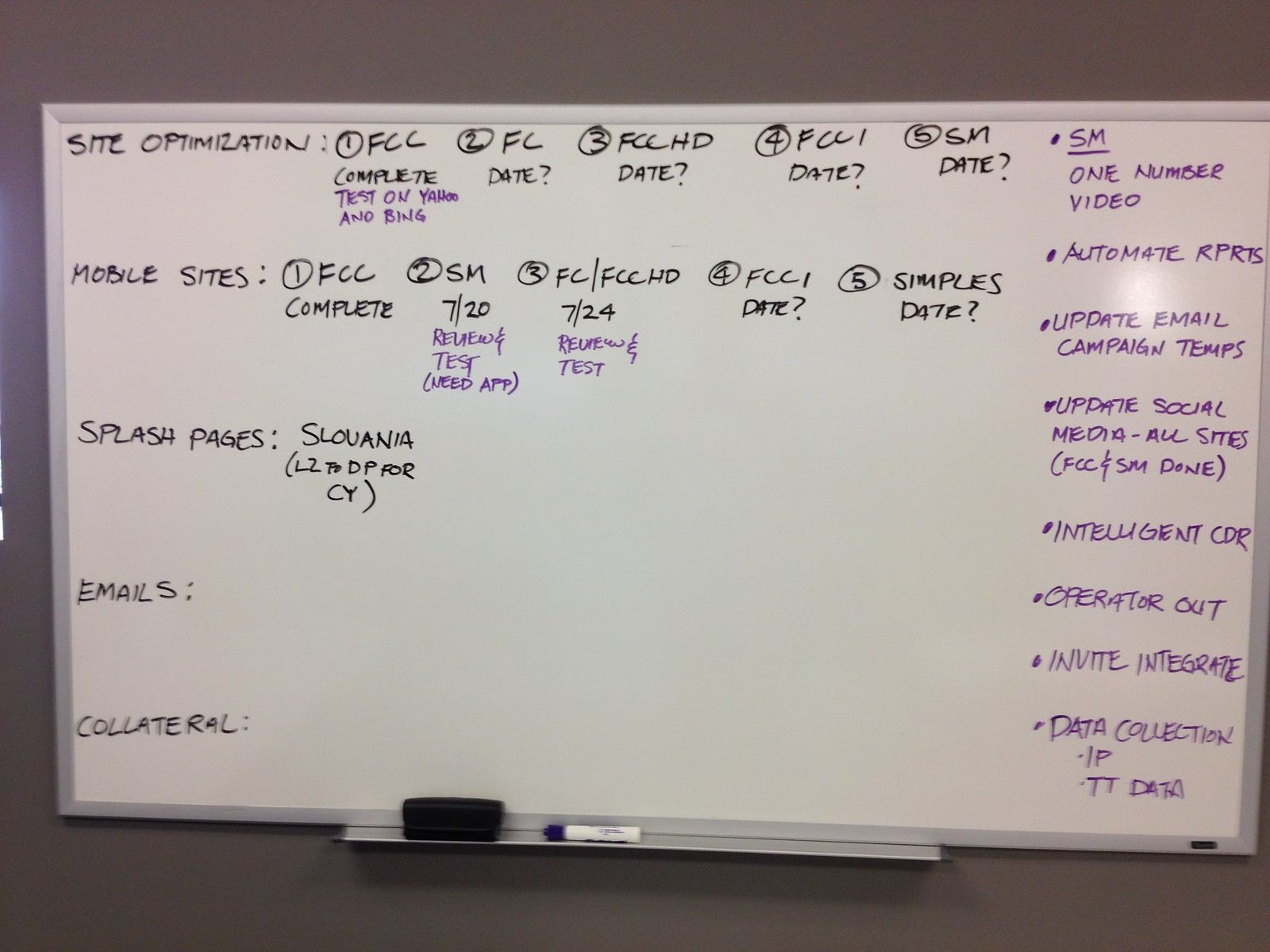In the image, we see an indoor setting featuring a rectangular whiteboard with a thin, silver metallic border, mounted on a tan wall. The whiteboard is filled with handwritten text in both black and purple marker. On the metal ledge at the bottom, there is a black eraser and a purple-capped marker.

The primary black text on the whiteboard is organized into a structured list. At the top left, the title "Site Optimization" is prominently displayed. Underneath, there are numbered points with specific entries: 
1. FCC - Complete
2. FC - Date?
3. FCC HD - Date?
4. FCC I - Date?
5. SM - Date?

Below this, another section titled "Mobile Sites" lists similar numbered points:
1. FCC Complete
2. SM 7/20
3. FC-FCC HD 7/24
4. FCC I - Date?
5. Symbols - Date?

Further down, headers for "Splash Pages," "Emails," and "Collateral" are displayed, although the "Emails" and "Collateral" sections are not filled out. Next to Mobile Sites, in purple ink, notes such as "Review and Test," "Need app," and "SM 1 video number" are presented, indicating task details.

On the far right-hand side, more detailed tasks are written in purple ink, such as:
- SM Automate Reprints
- Update Email Campaign Temps
- Update Social Media for All Sites (including FCC and SM)
- Intelligent CDR
- Operator Out
- Invite Integrate
- Data Collection IP TT Data

The image provides a comprehensive view of a whiteboard used for project management and task tracking with a focus on site optimization activities.